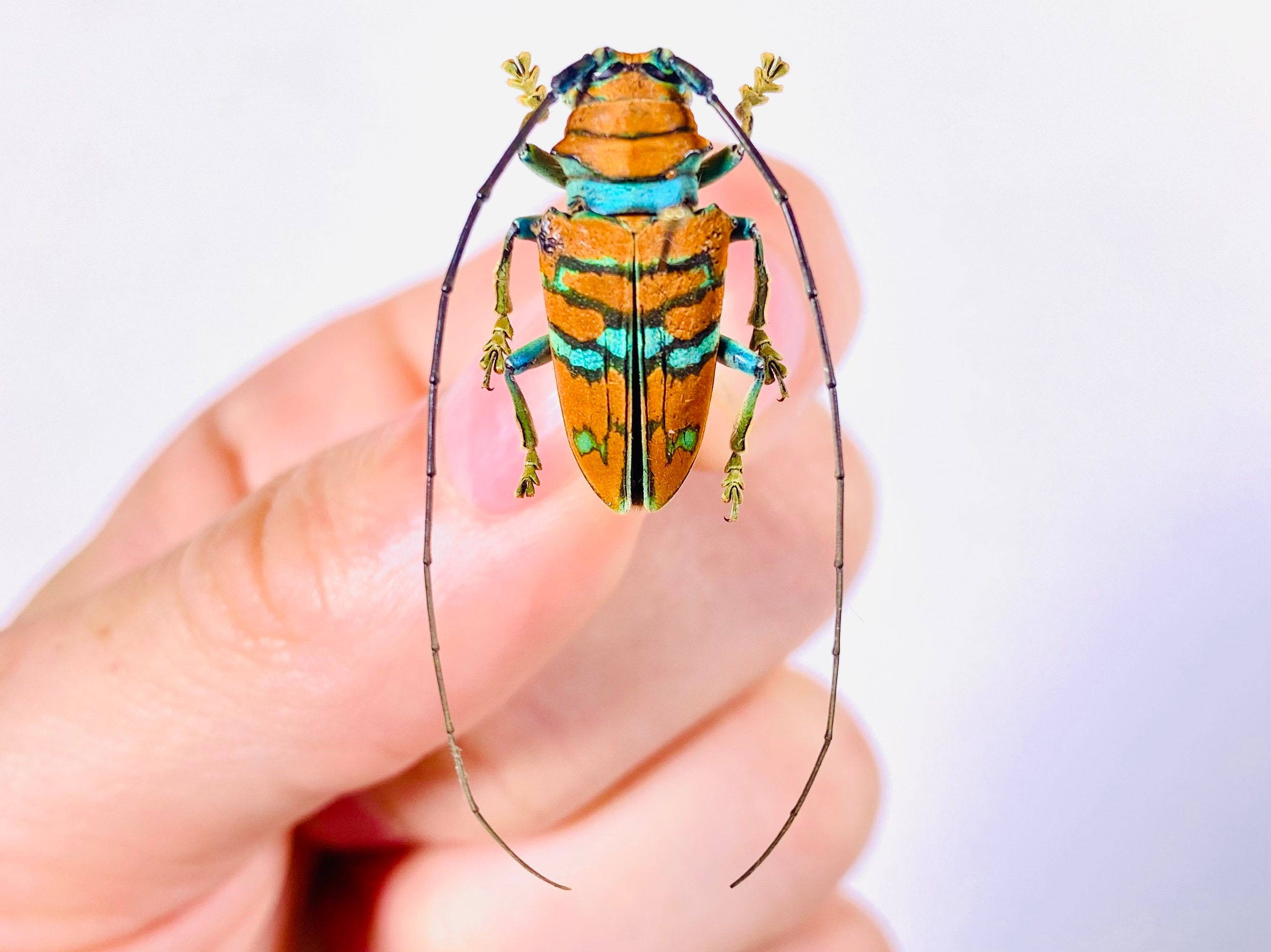In a sharply detailed photographic image set against a plain white background, a left hand with fair skin is carefully holding a striking insect between the thumb and index finger. The insect, a vibrant blend of orange and turquoise blue with some black bands, displays a striking pattern along its body. Its six legs are a mix of blue and brown, while a set of impressively long antennae, extending in an upside-down U shape from its head to beyond its body, add to its distinctiveness. From this close-up view, the turquoise band separating its head from its wings and body is clearly visible. The insect’s delicate wings, numbering two, are subtly visible, emphasizing both the intricate beauty of the creature and the precision of the hand that holds it.